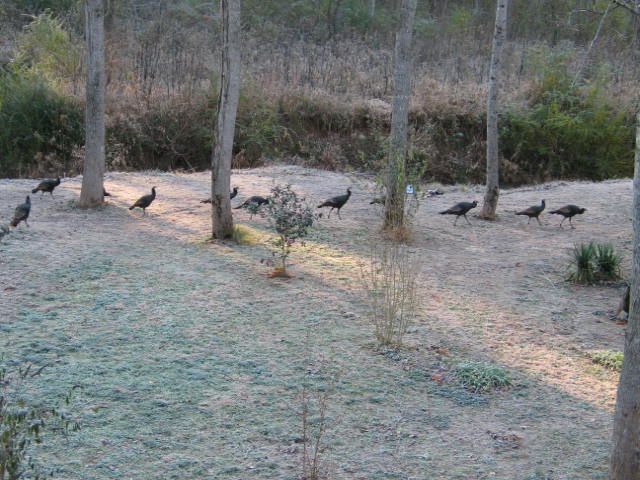In this grainy, low-light wildlife photograph, a group of nine or ten medium-sized black birds with long legs are seen walking along the dry, dull grass. The landscape appears lifeless, with the grass either frosty or dead, punctuated with small patches of vegetation that might be bushes or weeds. The scene is dominated by five slender, barren tree trunks positioned in a near-straight line, casting elongated shadows across the ground. The backdrop features sparse greenery, including bushes and small trees, enhancing the impression of a dry, almost desolate area. A streak of sunlight penetrates the scene from the top left, creating a strip of light that extends to the bottom right, subtly illuminating the somber, grayish tones of the image.